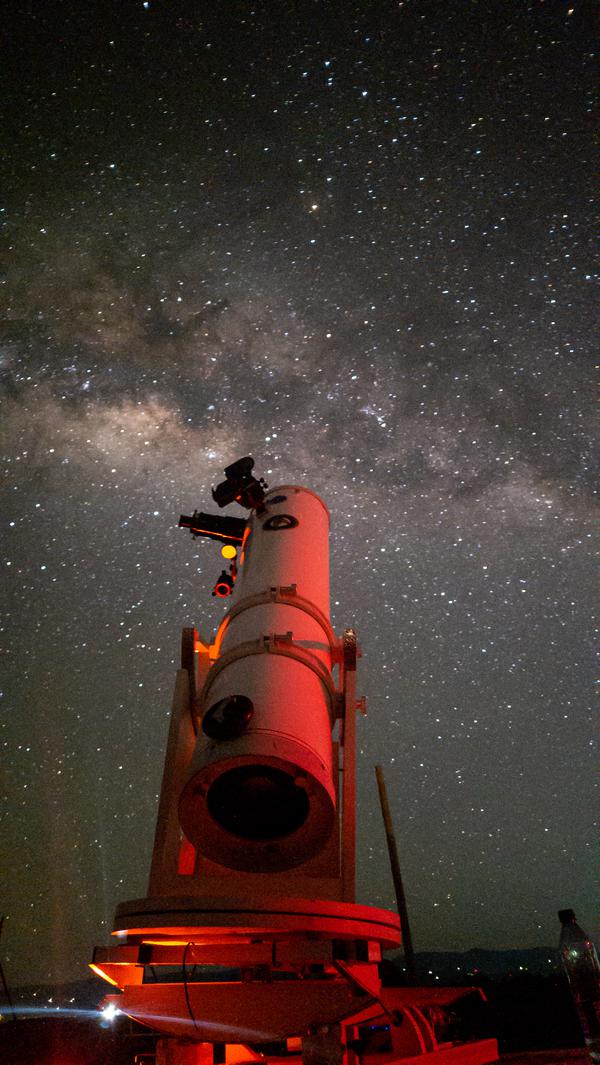This photograph showcases a large reflector telescope positioned prominently in an observatory setting. The telescope, a substantial piece of equipment often associated with serious astronomical research, is mounted on an automated fixture, indicating its likely use in a professional environment such as a college or university. The telescope itself is primarily white but is bathed in a red light, giving it a distinctive glowing appearance. Its long tubular structure, complete with prominent metal receptacles and a circular base also illuminated in red, suggests a sophisticated design aimed at high-precision observational work.

The night sky above is breathtaking, dramatically lighted by both a dense field of stars and the luminous band of the Milky Way galaxy, which stretches across in hues so intense that they render the sky more gray than black. There is a notable contrast between the darker upper portion of the sky and the lighter, almost mist-like sections below, possibly indicative of star clusters or interstellar gas clouds. The photograph appears to be a long-exposure shot, capturing the fine details and ethereal glow of the celestial landscape.

Details such as the eyepiece at the telescope’s far end and the additional fixtures on top illustrate the complexity of the instrument. The light attached to the side, likely used for adjustments, adds a functional touch to the scene. Despite the advanced equipment and detailed environment, the lack of people in the image highlights an isolated, serene moment of scientific observation. The distant bright light and small details like a water bottle contribute to the ambience, underlining the meticulous and immersive nature of stargazing.

In summary, this image eloquently captures the intersection of human technological achievement and the vast, awe-inspiring expanse of the cosmos, all framed within the soft, captivating glow of red light and the grandeur of a star-studded sky.